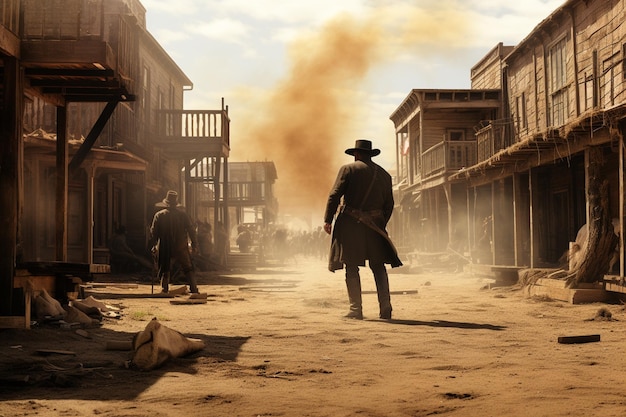The image, titled "Two Gunslingers at High Noon," vividly depicts a dramatic Western movie scene set on the dusty, dirt-covered main street of an old western town. Flanked by two-story wooden buildings with porches, wooden railings, and stairways, the street is strewn with debris, including rocks, boulders, and bits of sagebrush. The atmosphere is thick with a reddish-brownish smoke cloud that engulfs the background, partly obscuring the old wooden facades. In the center of the image stands a lone gunslinger, his back to the viewer. He is dressed in a long trench coat, knee-high boots, and a flat-top cowboy hat, with his hand poised on a gun, suggesting a potential shootout. Further down the street on the left, partially shrouded by the dust cloud, is another gunslinger wearing darker clothes and a larger, floppier cowboy hat. This man also appears ready for confrontation, with a gun visible on each hip. The overall scene is framed in dark, dusty hues that enhance the tension and the quintessential Wild West atmosphere.